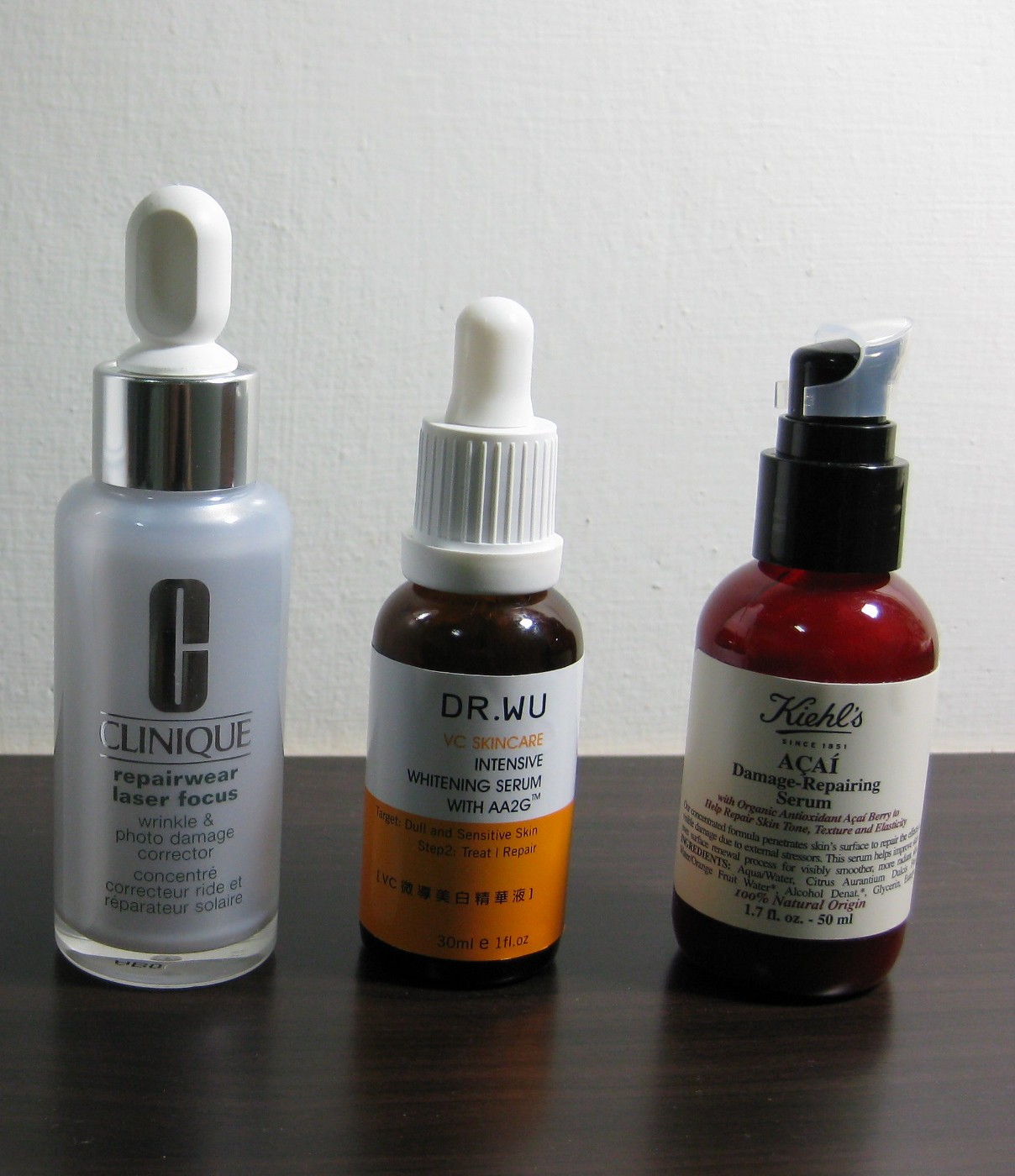A detailed caption for the given image could be:

"Set against a plain white wall, three skincare products are displayed on a dark tabletop. The lineup begins with Clinique's Repairwear Laser Focus Wrinkle & Photo Damage Corrector in a sleek, silver-gray bottle on the left. In the center, an amber bottle adorned with a white and orange label houses Dr. Wu's VC Skin Care Intensive Whitening Serum with AA2G, which includes notes on its suitability for sensitive skin alongside some text in what appears to be Chinese. On the right, a reddish-amber bottle stands out, containing Kiehl's Acai Damage-Repairing Serum, although the finer print details are too small to decipher. The clean, minimalist backdrop emphasizes the diverse packaging and branding of the products."